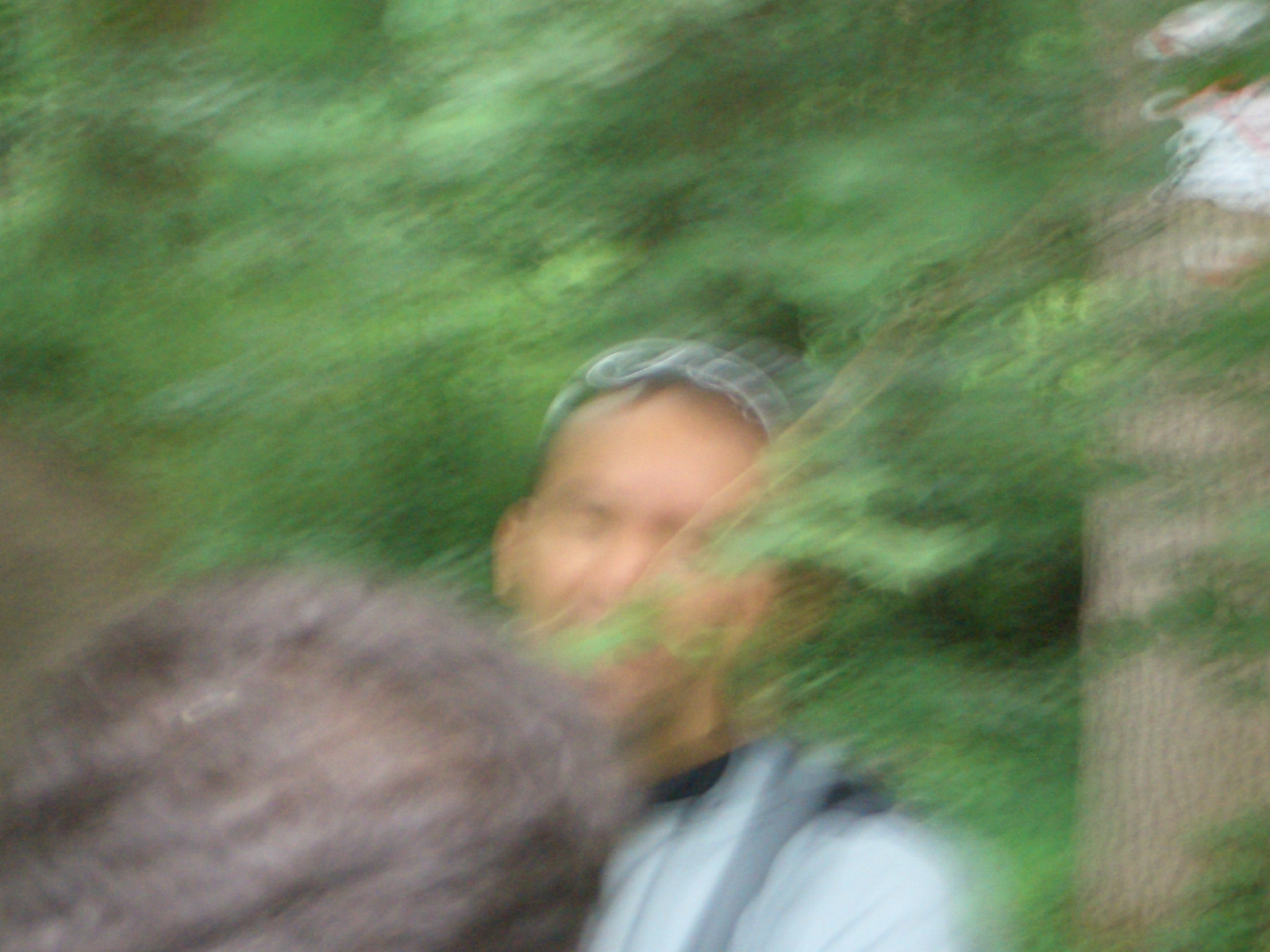This extremely blurry photograph depicts a Caucasian man, possibly outdoors in a forest or garden setting. He is the central figure, seen from his bicep upwards, and appears to be carrying a young tree. The tree is in front of his face, with small branches and green leaves partly obscuring it. The man is wearing a white jacket with a grayish hood draped down and has sunglasses pushed up on his head, revealing a wisp of brown hair. Behind him, a large tree and its trunk dominate the background. There's also a noticeable, very blurry blob of brown at the bottom left corner, likely representing a large clump of soil mixed with roots and grasses, suggesting the tree he is carrying is ready for planting. The overall lush, green setting indicates a natural outdoor environment.